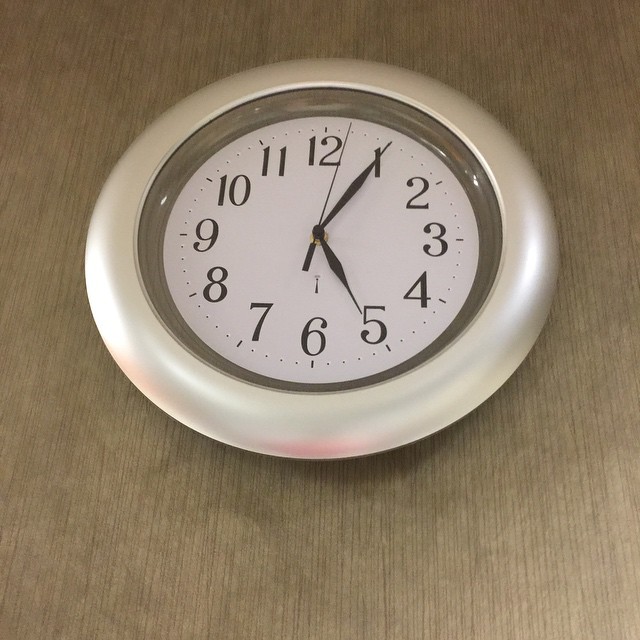A detailed indoor photograph captures a wall clock mounted on a light wood panel. This silver-bezel clock features a stark white face adorned with black numerals ranging from 1 to 12. The time indicates 5:05, with the black second hand pointing just past the 12, precisely at the 2-second mark. The clock appears brand new, showcasing a clean, unmarked surface devoid of any text or branding. The photograph is taken from a slight upward angle, making the bottom of the clock more prominent in the frame while the top recedes into the background. The face of the clock is shielded by a plastic cover, contributing to the clock's overall plasticky appearance. The lighting in the image is slightly brighter at the bottom, adding subtle contrast to the scene. Despite its pristine condition, the clock has an inexpensive look, suggesting it is a budget-friendly model.